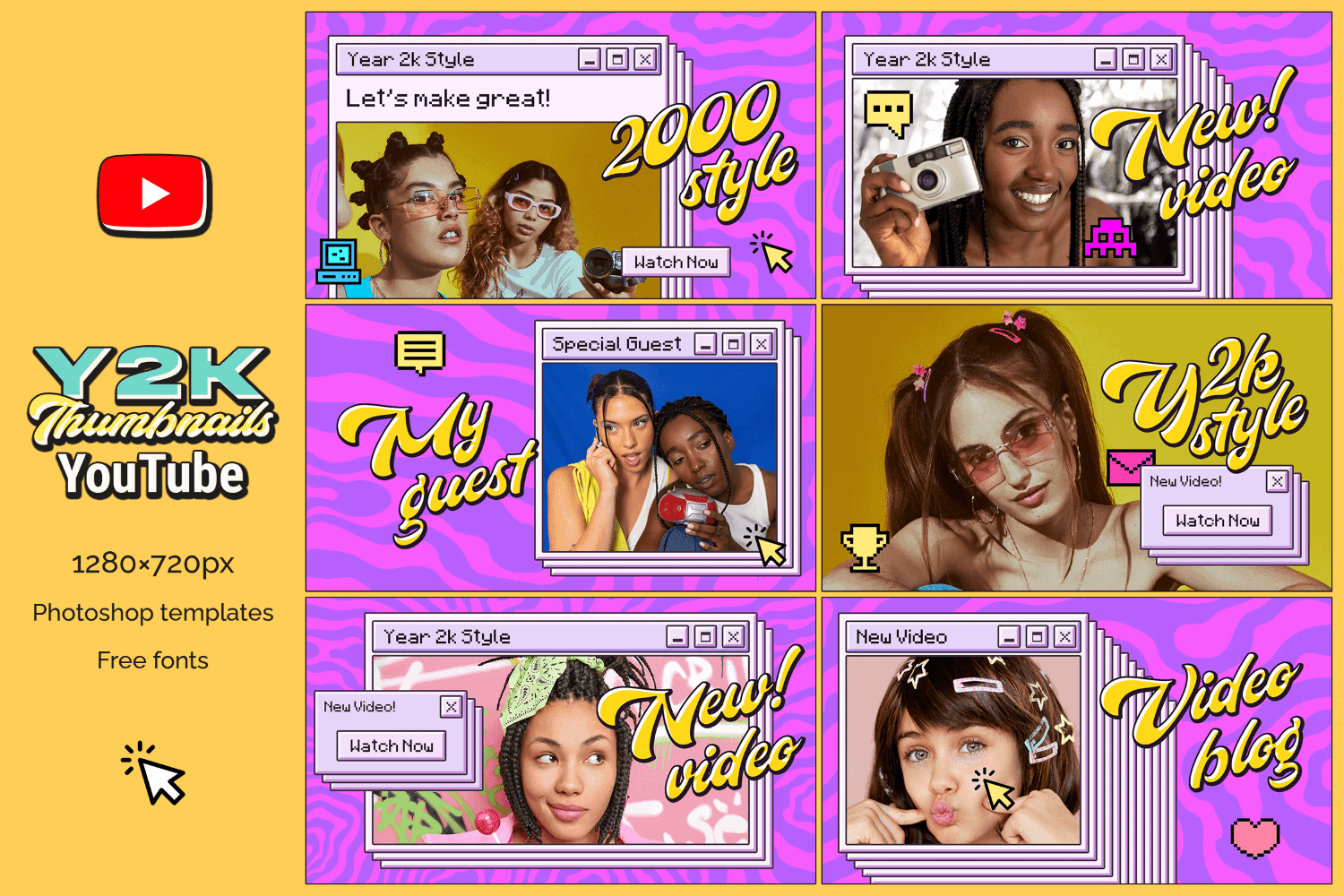This image features a vibrant, Y2K-themed YouTube Thumbnails template, set against a striking yellow background. The central visual element is a red button with a right-pointing arrow. The template dimension is 1280x720 pixels and includes free fonts. A prominent white arrow with dashed lines adds a dynamic effect.

Six images showcase various Y2K styles:

1. **Year 2K Style**: Features a girl with braids all over her head and oversized glasses, with another girl who has long, flowing hair. The scene is set against a purple and pink wavy background.
  
2. **My Guest**: Displays two girls together; one wearing a Starburst-themed shirt. Both are set against the same purple and pink wavy background.
  
3. **Year 2K Style, New Video**: Shows a girl with a stylish bow scarf tied in her hair, holding a lollipop.
  
4. **Y2K Style, New Video**: Features a girl with dreadlocks holding up a camera.

5. **Y2K Style**: This image, set against a yellow background, shows a girl wearing glasses and sporting pigtails.
  
6. **New Video Blog**: Highlights a girl with short hair and bangs, pointing to her dimples with her fingers.

Each thumbnail is meticulously designed to capture the essence of the Y2K era, making them perfect for retro-themed content.